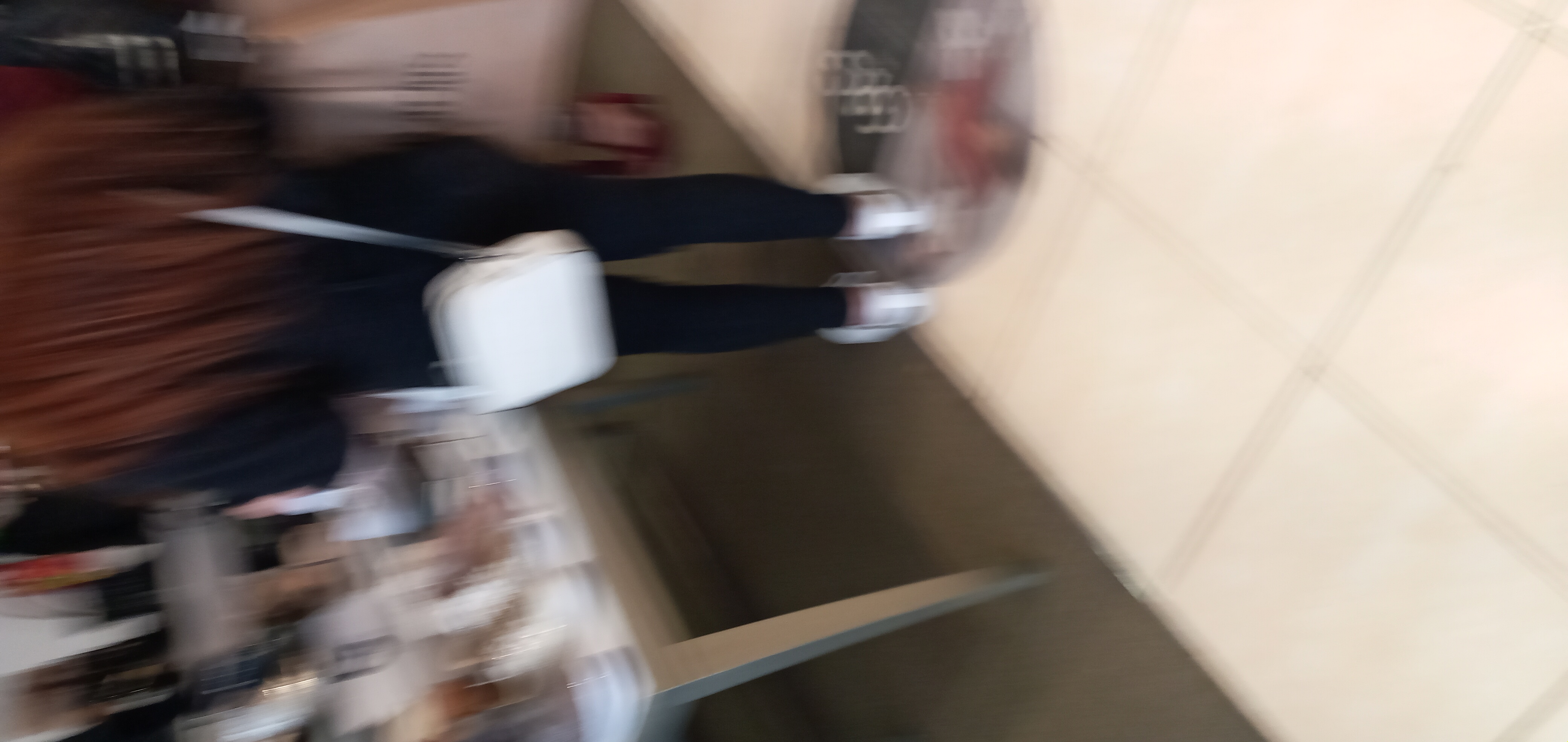This horizontally rectangular, extremely blurry photo appears to have been taken with the camera in significant motion, resulting in a low-quality, shaky image. The photo needs to be rotated counterclockwise to be properly viewed. It captures the backside of a young woman with long auburn or reddish-brunette hair, wearing a black top, dark black or blue tight-fitting pants, and white shoes. The woman also carries a white crossbody purse that drapes over her shoulder and covers her buttocks. The setting seems to be inside a store, potentially a department or cosmetic store, as suggested by the visible large, square white tiles on the floor and a table filled with indistinguishable items due to the blur. The scene further includes a section of darker flooring, possibly carpeted, and a sense of looking downward at an angle, which adds to the disorientation caused by the image's rotation.